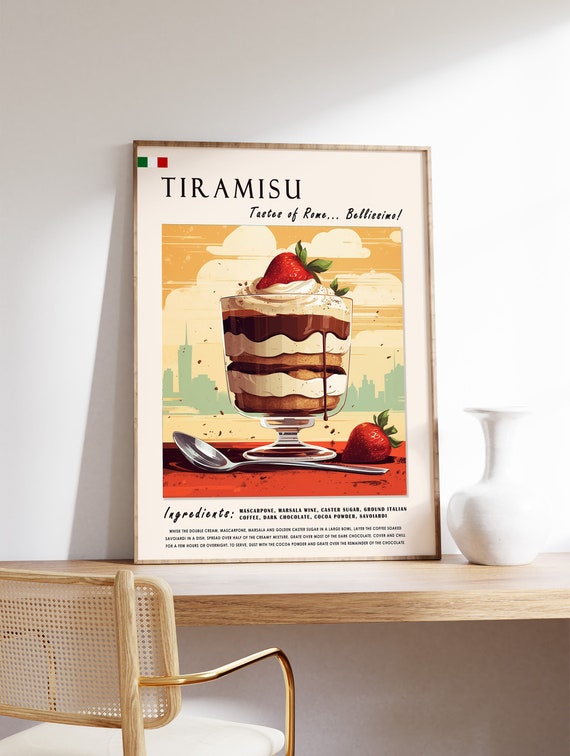The vertical rectangular poster of tiramisu rests on a light blonde wooden surface, seemingly built into the wall. The table features a chair with a matching blonde wood back, white cushion, and elegant gold armrests, positioned facing the table. The poster is adorned with the striking text, "Tiramisu: Taste of Rome, Bellissimo!" prominently at the top. It showcases an intricate drawing of tiramisu in a parfait dish, layered with rich chocolate, tan cake, and fluffy whipped cream, all topped with whipped cream and a strawberry, with an additional strawberry's leaves visible. The dessert sits on a vivid red surface, accompanied by a silver spoon and another strawberry positioned beside it. To the poster's right is a sleek white vase, round at its base with a flared top, adding a touch of elegance to the scene. The entire image is a masterful blend of culinary arts and tasteful décor, capturing the essence of a delicately designed space.